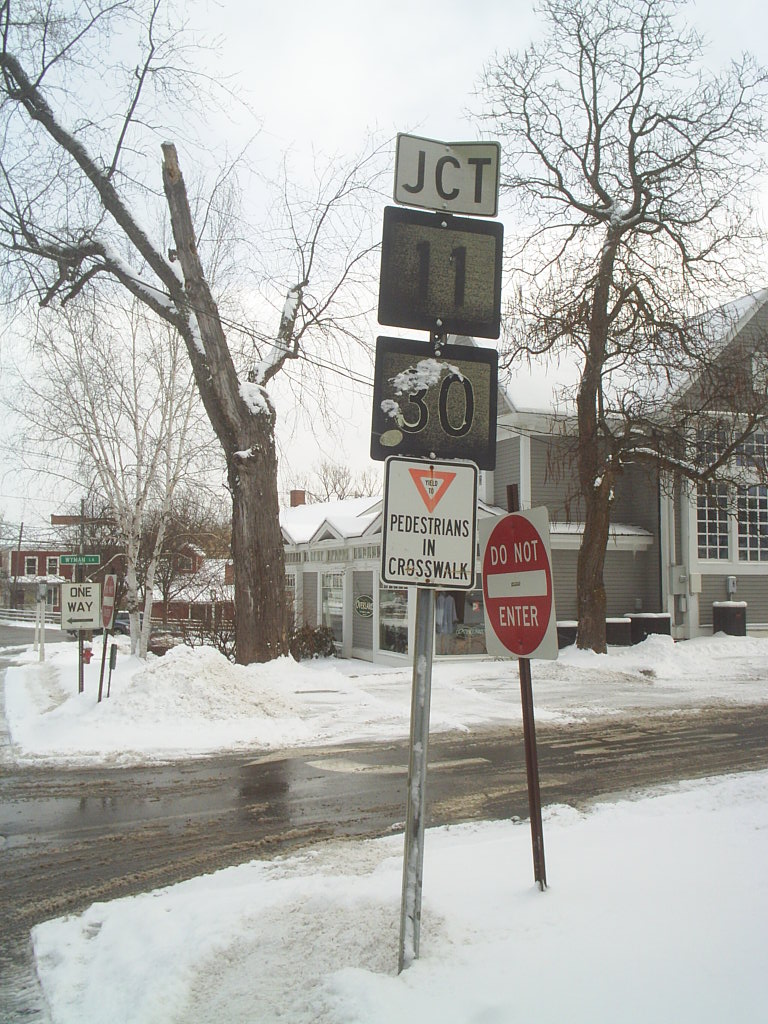A serene, snowy outdoor scene is captured with several distinct elements. Prominently in the foreground, there is a signpost adorned with multiple signs: a red triangle cautioning pedestrians and indicating a crosswalk, topped with "30" denoting a speed limit, and a smaller sign labeled "JCT" at the very top. Below that, there's a "Do Not Enter" sign represented by a red circle with a white rectangle in the center. To the left of the signpost, another sign directs traffic "One Way," pointing left. A green sign also appears among the collection. The ground is heavily covered with piles of pristine white snow. Bare, dormant trees with brown branches stand against the wintry backdrop, their stark silhouettes contrasting with the expansive white sky.